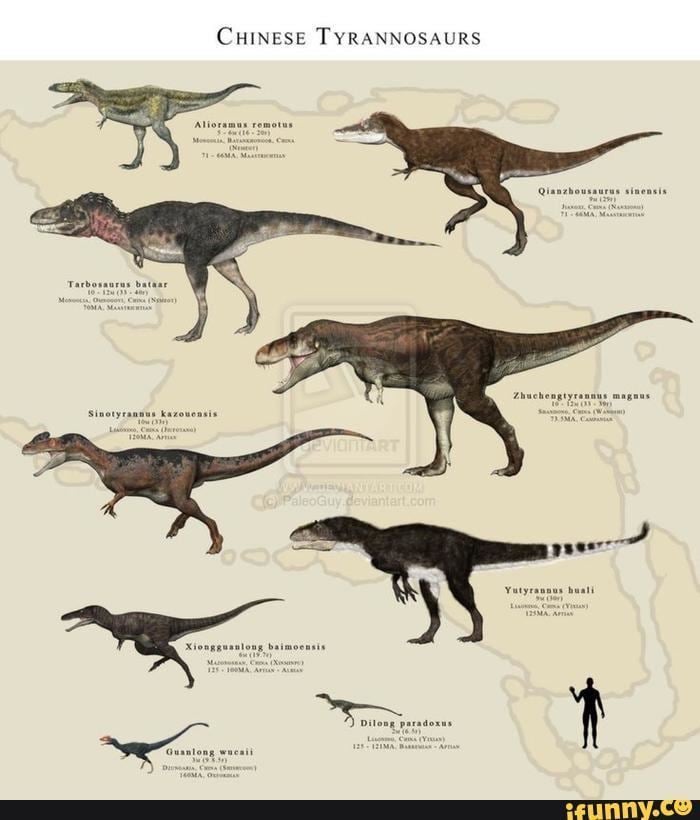In the image, a detailed educational poster titled "Chinese Tyrannosaurus" is displayed prominently at the top. The poster features a beige background resembling a map of a specific area, possibly an island surrounded by water. There are nine distinct dinosaurs illustrated in various sizes and colors, each labeled with scientific names and additional information that is too small to clearly read. 

In the upper left corner is a small dinosaur named Alaramis Remotus, distinguished by its green body, short arms, long legs, and a light-colored stomach. Directly below it is a larger dinosaur, Tarbosaurus Bataar, notable for its long tail, purple neck hump, and lighter-colored stomach and legs. 

In the upper right corner is a medium-sized, darker brown dinosaur with white under its face and stomach. Moving to the lower sections, in the middle of the page is the largest dinosaur in the poster, characterized by a wide-open mouth, dark brown color, and light underbelly and inner legs. 

To the bottom left of this large dinosaur, there's a smaller one with a distinctive bill on its nose, adorned in red, brown, and black. Below this, leaning forward, is a nearly black dinosaur with a light face and several white stripes on its tail. 

Further to the left is a very small, dark-colored dinosaur. Extending to the far bottom left corner is another tiny dinosaur, red-billed, dark gray in color, with a curled-up tail. In the lower right corner, a figure of a man, shaded in black, is shown with his arm raised, likely for scale comparison with the dinosaurs. The entire poster is framed with a black border at the bottom, bearing the watermark "ifunny.co" with a smiley face inside the "O."

The dinosaurs are arranged in a zigzag pattern across the poster, and despite the text being hard to read, it includes details such as their names, sizes, origins in China, and potentially the historical periods they belonged to. The overall color scheme features black, tan, gray, brown, orange, red, and yellow, contributing to the scientific and educational aesthetic of the poster.